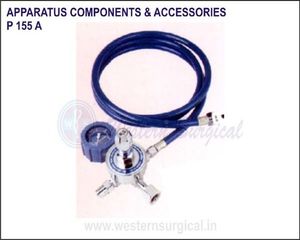The image shows a blue coiled hose with multiple attachments and nozzles for a different apparatus, alongside a pressure gauge. The hose is attached to a central silver valve with various outlets. The image has a white background and a thin dark blue-black outline. At the top in navy blue font, it reads "Apparatus, Components and Accessories" followed by the part number "P155A." The branding of "Western Surgical" is overlaid very translucently across the image, and at the bottom, the web address "www.westernsurgical.in" is displayed. The hose setup features a pressure gauge on the bottom left portion, indicating its functionality in measuring pressure.